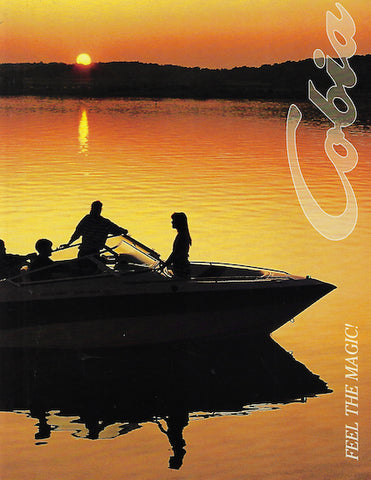This advertisement for Cabo captures the mesmerizing beauty of a sunset over a calm lake. The small, vertical rectangular image is dominated by warm hues of gold, orange, and yellow radiating from a golden-orange sun setting slightly above a tree-lined, hilly shoreline. This picturesque backdrop serves as a canvas for a small motorized family boat, silhouetted against the glowing water. The boat, with its modern design and outboard motors, reflects gracefully on the lake's shimmering surface. In it, we see the silhouettes of four people: a woman standing at the front gazing back toward three gentlemen, one of whom is standing at the helm steering the boat. The scene exudes tranquility and adventure, encapsulated by the vertical white text on the right side that reads, "Feel the Magic," and a watermark on the top right proclaiming "Cabo" in semi-transparent cursive letters. The entire image is suffused in rich shades of orange and gold, creating an inviting and magical atmosphere perfect for a travel advertisement.